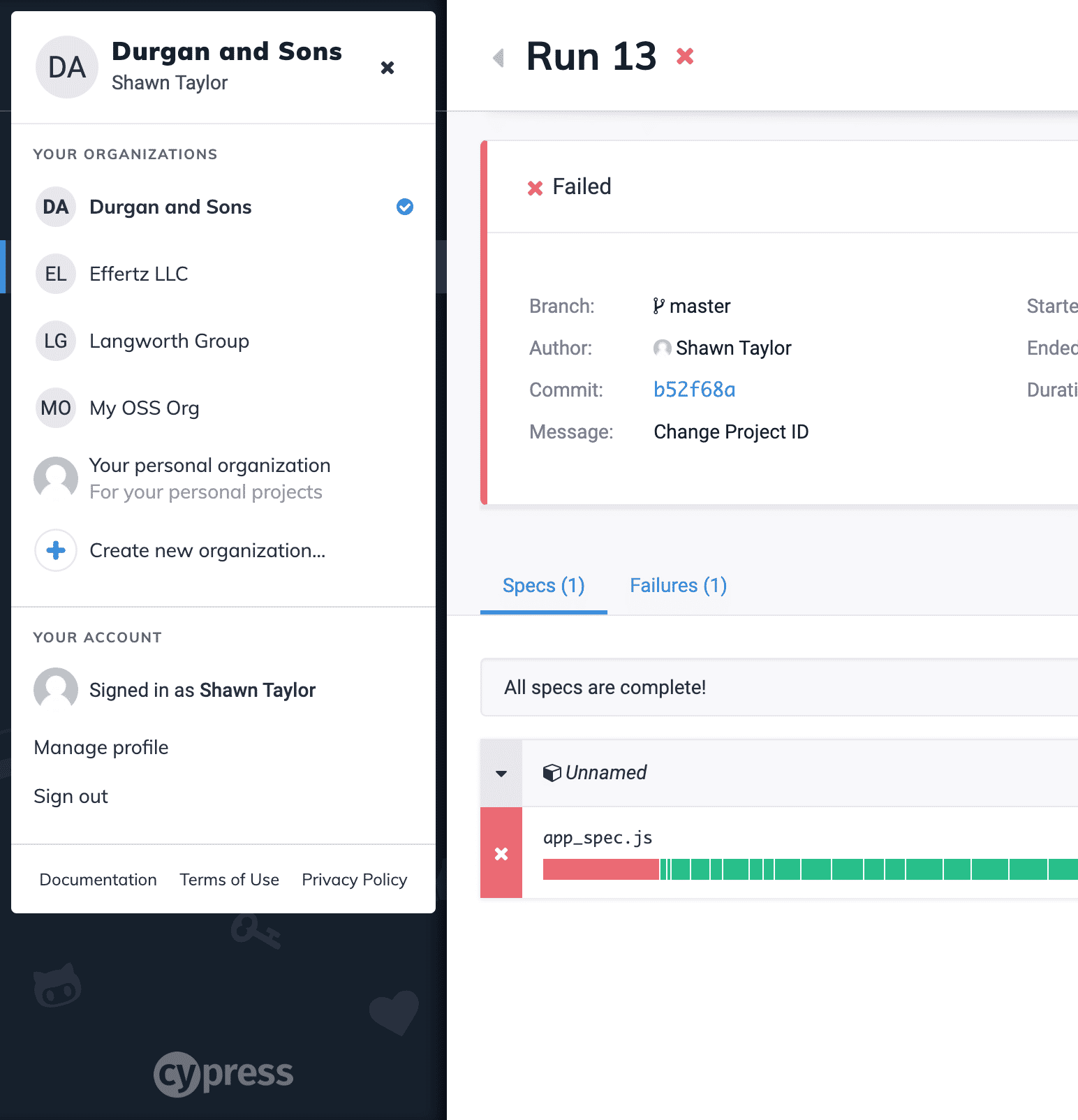**Descriptive Caption:**

In this image, there are two separate windows displayed side by side. The first window, positioned on the left, is titled "Durgan Incense" and shows the user Sean Taylor's profile. Below the title, a list of different organizations associated with the user is displayed in sequential order: "Durgan Incense," "Ifritz LLC," "Langworth Group," and "MyOSS.org." The bottom section of this window provides a brief description of Sean Taylor's account, including options to manage his profile or sign out. At the very bottom, there is a logo for "Cypress," featuring the letters "C" and "Y" inside a dim light gray circle.

The second window, positioned on the right, appears to be a computer terminal or software interface. It has a header labeled "Run 13" and contains a message log. The log identifies "Veiled Branch Master, author Sean Taylor," along with a commit identifier "B52F68A." The message detail indicates a change made to the project ID.